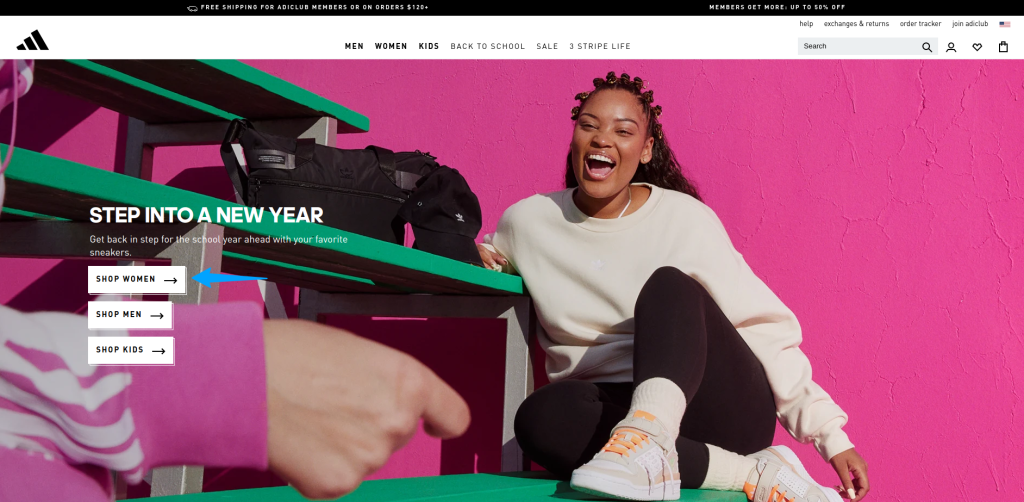Screenshot from the Adidas website showcasing a vibrant and engaging layout. At the top, a sleek black border is followed by a white navigation bar featuring categories: Men, Women, Kids, Back to School, Sale, and Stripe Life. On the right, there's a search bar, a heart icon, and a shopping bag icon.

Dominating the center is a striking photograph set against a pink background. An African American woman with cornrows, dressed in black pants and a tan sweatshirt, sits casually on green bleachers. She sports stylish tan shoes with orange laces and has an open, joyous smile. A pink-and-white tracksuit-clad arm is partially visible from the bottom left, adding a dynamic element to the scene.

On the left side of the image, bold text reads "Step into a new year," accompanied by three white buttons labeled Shop Women, Shop Men, and Shop Kids, with a blue arrow pointing to the Shop Women button.